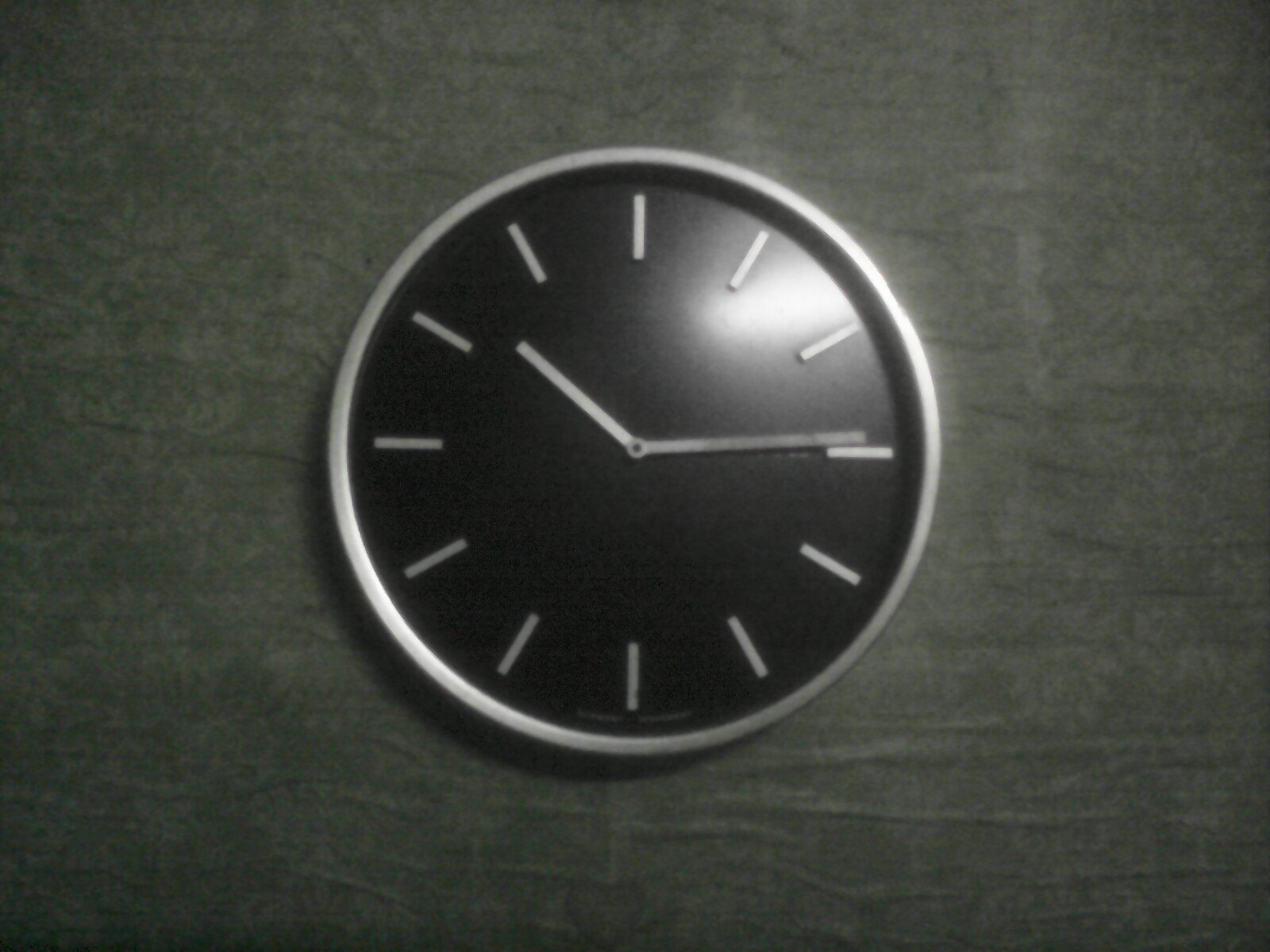The image portrays a sleek, modern clock mounted on a textured, dark gray wall. The clock occupies the center of the composition, standing out due to its minimalist design. The clock's face is primarily black, accentuated with a silver trim that adds a touch of sophistication. Instead of traditional numbers, stainless steel markers indicate the hour positions, and both the hour and minute hands are made of the same polished metal, enhancing the clock's contemporary aesthetic. A soft reflection on the clock's glass face suggests ambient lighting from the room. The hands point to what appears to be 10:14, the absence of numerals requiring familiarity with clock reading to ascertain the time.